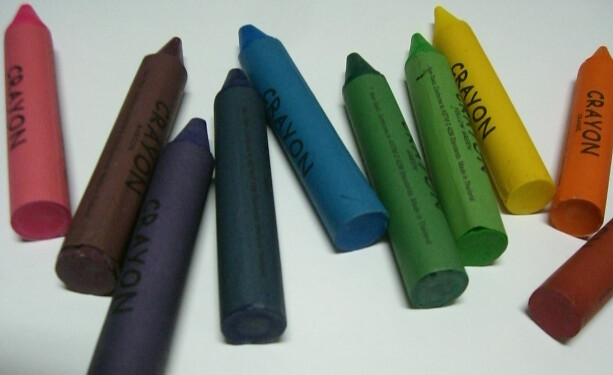In this photograph, a selection of short, generic crayons is arranged haphazardly on a light orchid background. The crayons, all pointing upwards, are laid side by side but in varying directions. From left to right, there is a pink crayon, followed by a brownish-gray, a deep purple, an indigo of deep blue, a medium blue, a dark green, a lighter green, a yellow, an orange, and finally, a red crayon, which is partially cropped out of the frame, revealing only its bottom half. Each crayon has a wrapper that matches its color, emphasizing their generic look without any prominent branding. While these crayons are notably shorter and possibly thicker than standard ones, they retain their vibrant, distinct hues.